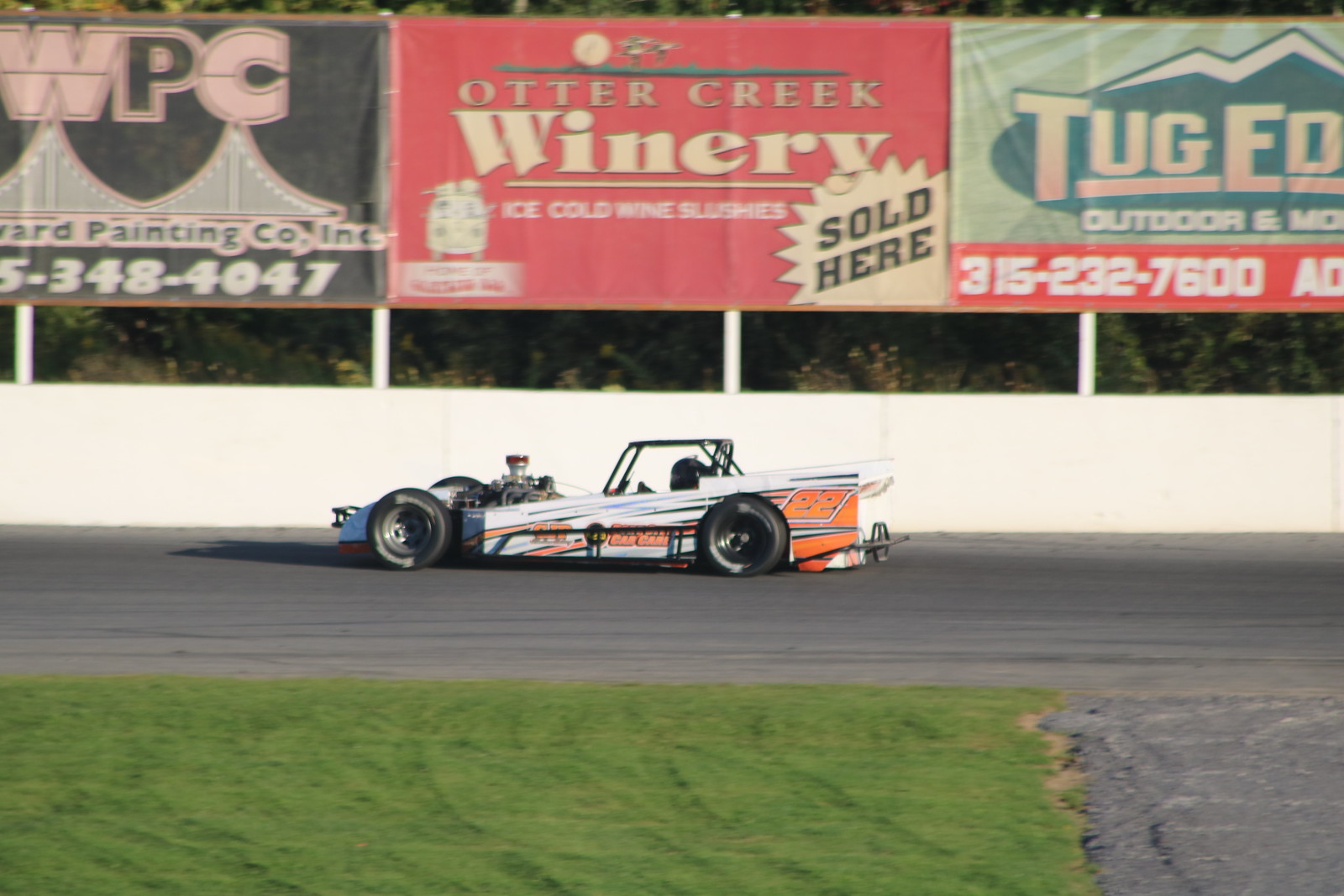This image captures a close-up of a vintage race car, distinctly numbered 22, navigating an asphalt racetrack. The car, reminiscent of models from the 1960s or 70s, features an exposed engine and an open cockpit showcasing the driver's helmet. Painted in a striking combination of orange, blue, and white, the race car sits low to the ground with a wedge-like shape and large black wheels. Surrounding the track, there's a narrow strip of grass and a patch of gravel likely intended for pit crews. Prominent in the background are three advertisement billboards attached to a white fence, supported by cylindrical poles. The advertisements promote a local painting company, Otter Creek Winery, and an outdoor store with a partially visible name where "Tug" is all that can be read. Behind these billboards, a line of trees and bushes is partially visible, framing the racetrack scene.